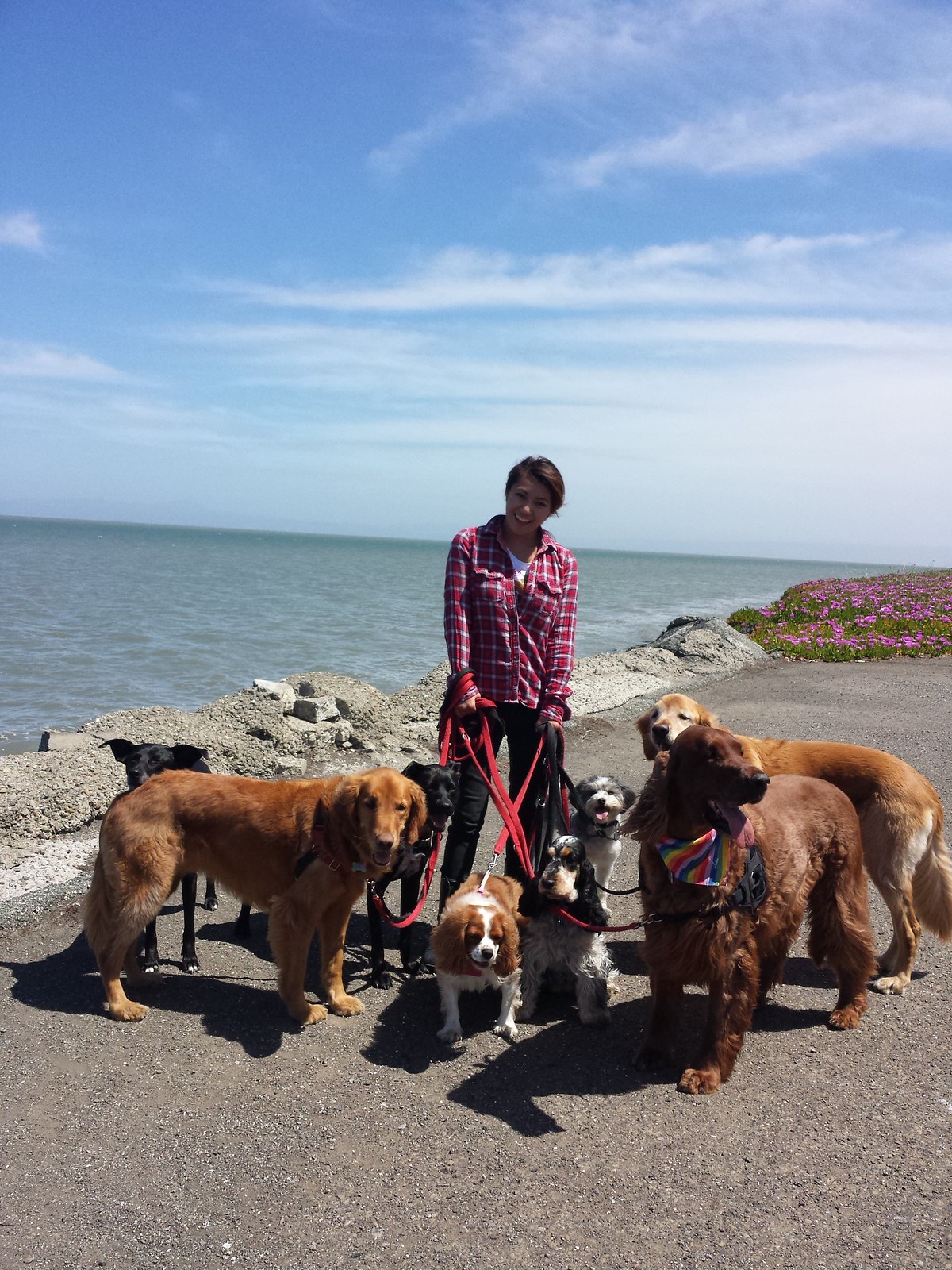Standing by a rocky beachfront, with the ocean's murky green waters and hazy blue sky as the backdrop, a woman is captured in the center of the photo, holding the leashes of eight diverse dogs. She is dressed in a red and white plaid lumberjack-style shirt over a white t-shirt, paired with blue jeans. Her medium-length hair is parted to the right. The leashes she holds in both hands are all uniformly red. The dogs she manages include three large ones resembling golden retrievers or red setters, three medium-sized dogs, and two small ones, including a Cavalier King Charles. She stands on the concrete, smiling brightly, effortlessly managing her pack of pooches on what appears to be a lovely day.